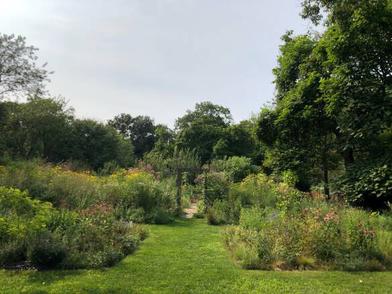This captivating photograph captures a serene garden scene with lush greenery and hints of vibrant colors. The focal point is a well-trimmed grass path that extends from the foreground toward a wooden archway, flanked by dense foliage and tiny purplish flowers on either side. The sky above is slightly overcast, casting a grayish-blue hue. In the background, a dense tree line creates a natural, enclosed atmosphere. Closer to the viewer, flowering plants and bushes add splashes of red amidst the predominantly green landscape. The setting evokes a peaceful, nature-filled environment perfect for a leisurely walk or a quiet picnic. Further beyond the archway, the grassy path transitions into a paved walkway, inviting one to explore deeper into this tranquil natural sanctuary.